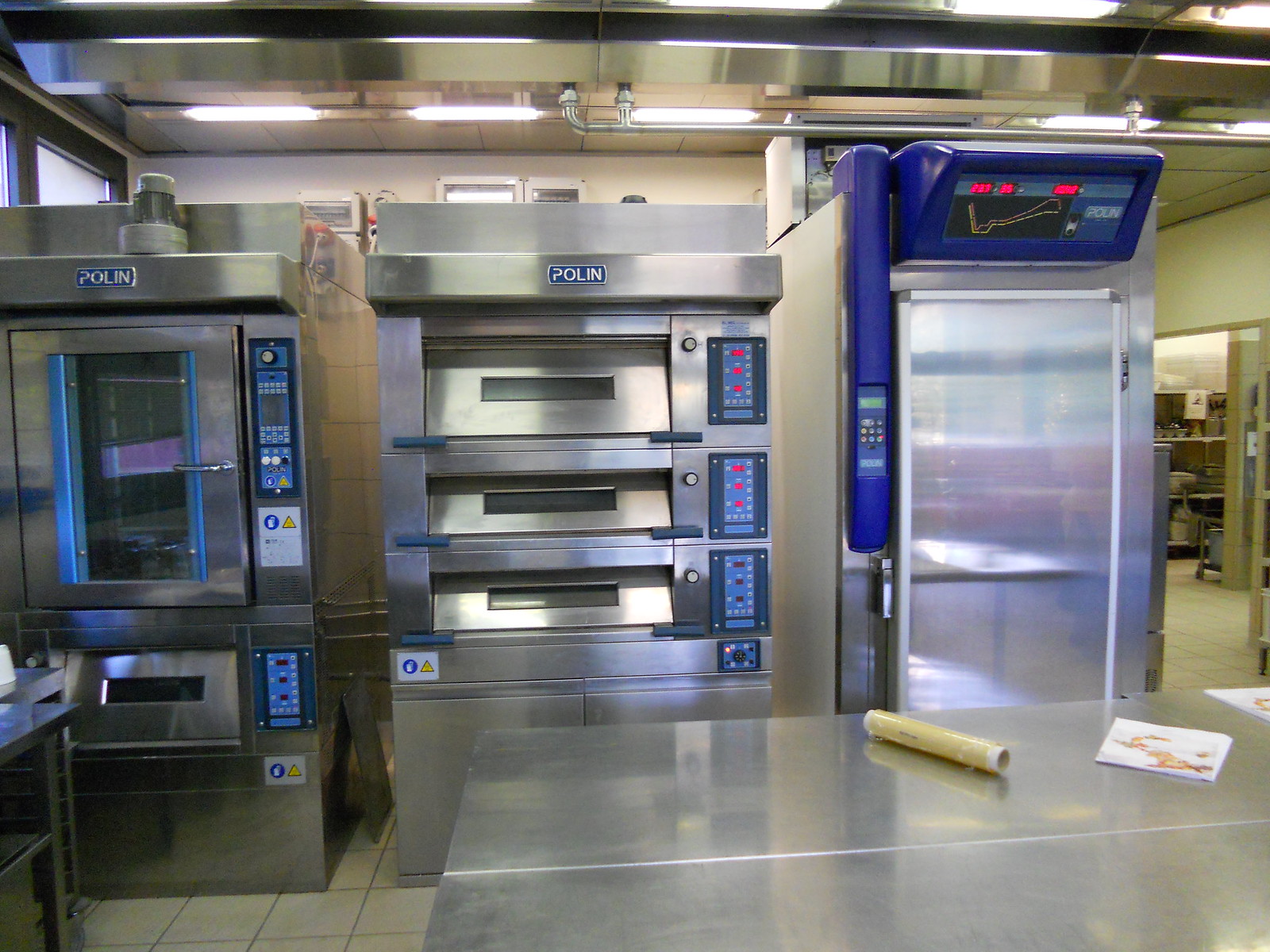The photograph depicts a commercial kitchen with industrial appliances, primarily made of stainless steel. In the foreground, a stainless steel table is visible, bearing a roll of saran wrap and some paper sheets with diagrams on them. The kitchen floor features white square tiles. Three large silver rectangular machines, larger than standard refrigerators, are lined up side by side with one-foot gaps between them. The machines all bear the brand name "Polin" at the top and possess control panels with blue backgrounds, buttons, and red LED displays. On the left, there is an upright oven with a clear window in the center of the door, potentially also serving as a proofer for bread. Multiple machines in the middle are likely pizza ovens, with their doors stacked vertically and equipped with pull-down handles. To the right, another large appliance, possibly a warming oven, features a refrigerator-like door. The kitchen ceiling is also metallic, equipped with recessed lighting and some visible pipes. In the background, cluttered shelves can be seen in an adjacent room, adding to the industrial atmosphere of the space.